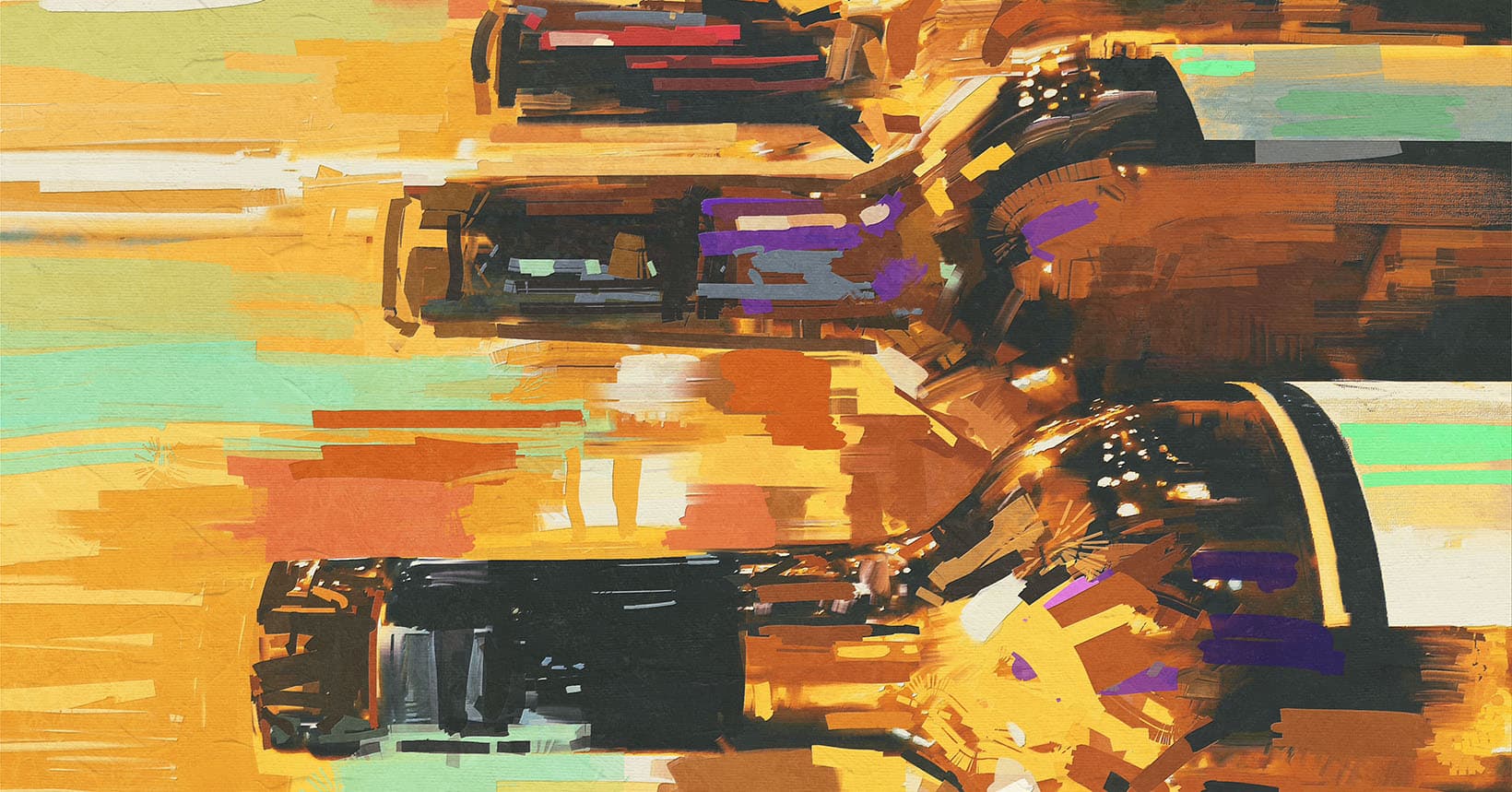The image is an abstract oil painting intended to resemble three wine bottles, presented in a bold and vibrant style. The bottles are displayed lying horizontally, side-by-side, showcasing their upper halves, including the cork necks and partially visible labels which are blank and unmarked. The color palette of the painting is dominated by rich shades of amber, brown, mustard yellow, and bright orange, with additional accents of mint green, turquoise blue, white, peach, black, and purple. The background mirrors this complexity, featuring an array of abstract blocks and bars of similar hues, enhancing the overall abstraction. The visible brushstrokes are thick and rectangular, creating a textured and layered appearance.